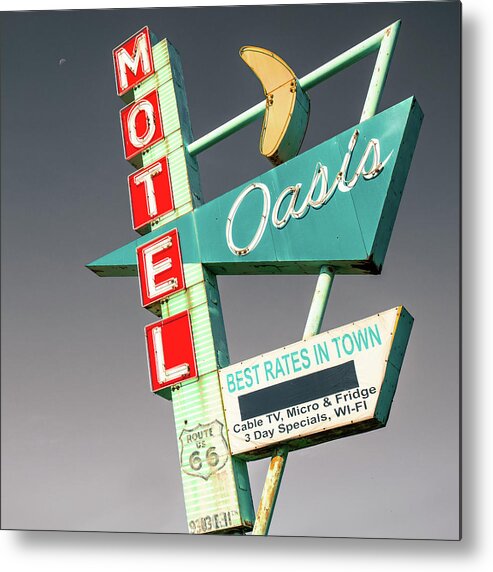This image features a retro-styled sign for a motel named "Oasis," prominently featuring a mix of green, red, and white colors accompanied by rustic brown hints due to some rusting. The unique design includes a vertically aligned, rectangular green sign with the word "MOTEL" written in white letters placed on red rectangles. An extending part resembling the number '7' arches out from the main sign structure. The highlight of the sign is a green triangle intersecting the larger rectangle, displaying the word "Oasis" in cursive. Additional text below offers essential details: "Best rates in town, cable TV, microwave and fridge, 3-day specials, and Wi-Fi." A reference to Route 66, "Route US-66," adds to the sign's nostalgic allure, evoking a 1960s motor hotel theme. The aesthetic is further enhanced by subtle yellow accents, completing the vintage vibe.